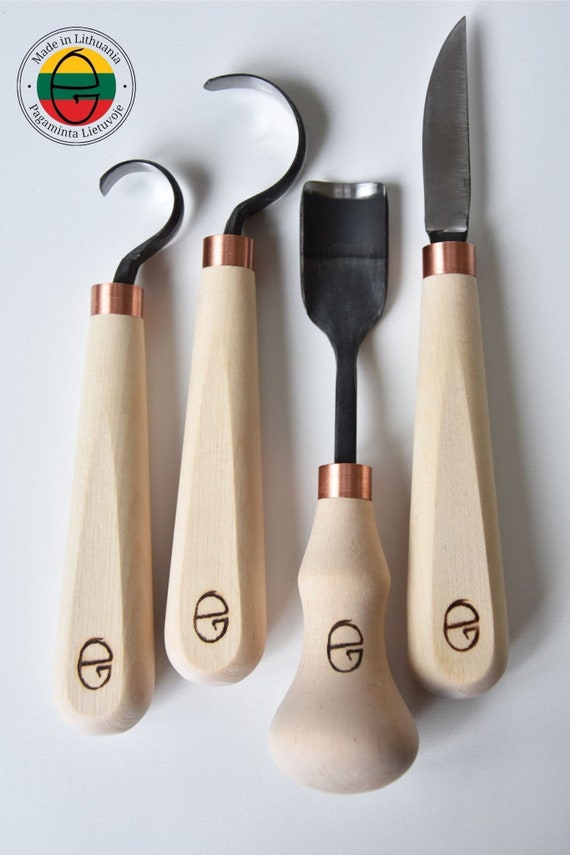The image features four hand tools arranged against a bright white background, providing clear visibility and detail. Each tool is equipped with a wooden handle accentuated by a bronze-colored collar near the tool's head. The handles display a distinctive logo: a stylized letter ‘E’ with a unique design indicating it might be from another language, most likely Lithuanian, as inferred from the "Made in Lithuania" text accompanying the logo in the top left corner of the image. This logo is set within a split circle that is green in the center, yellow on the top, and red on the bottom.

Two of the tools have hooked metal heads resembling the shape of a question mark, suitable for carving; the smaller hook looks sharper than the larger one. The third tool has a flatter, shovel-like head with curved sides and a sharp edge, and the handle ends in a knob. The fourth tool is a short knife with a pointed blade, featuring an extended handle similar to the hooked tools. Each tool exudes craftsmanship with its gold-etched branding, highlighting the attention to detail in their manufacture.